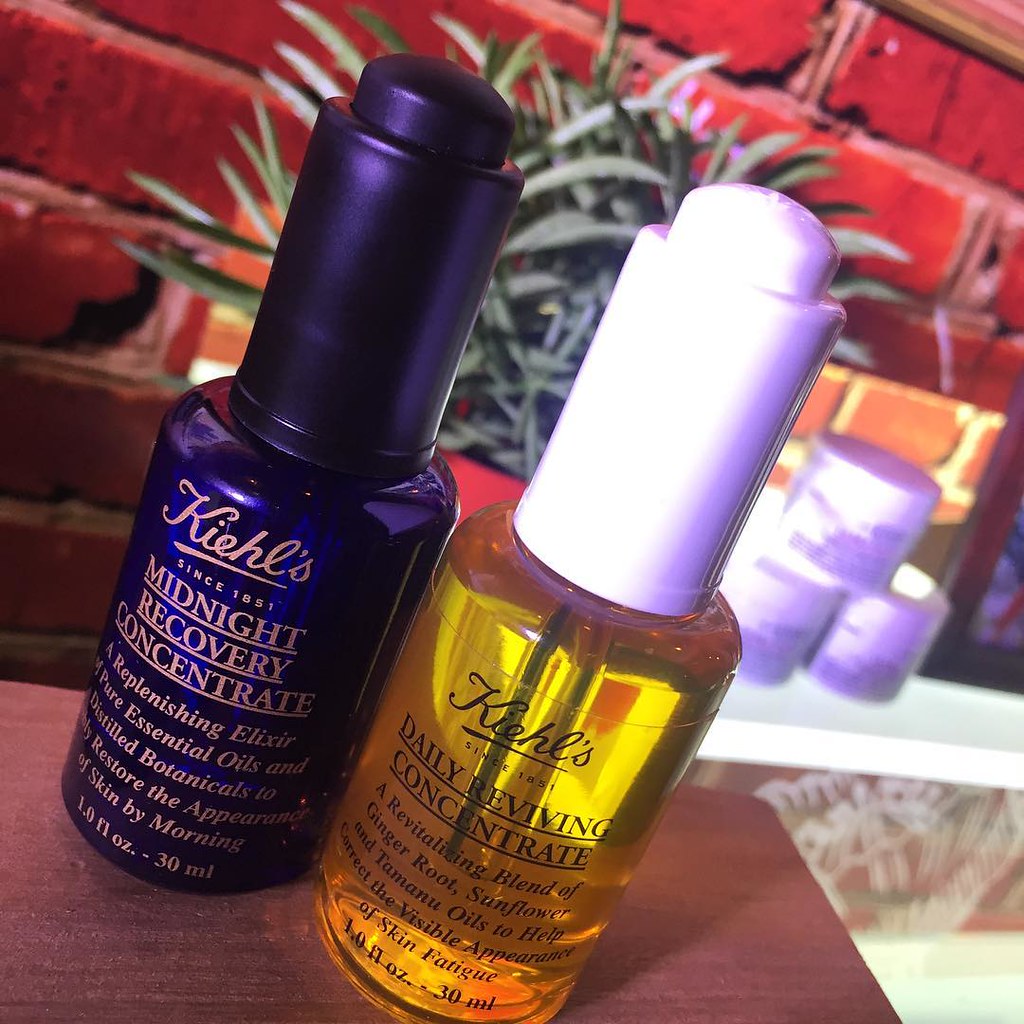This photograph showcases two Kiehl's beauty products sitting on the edge of a brown wooden table, positioned in front of a brick wall with a fireplace and an adjacent plant. The first product is the Midnight Recovery Concentrate, housed in a dark blue, nail polish-sized vial with a matching blue cap. The label describes it as a replenishing elixir made from pure essential oils and distilled botanicals, designed to restore skin appearance by morning. The second product is the Daily Reviving Concentrate, contained in a transparent vial with a white cap, filled with an orange-colored liquid. This product is a revitalizing blend of ginger root, sunflower, and tamarind oils aimed at combating skin fatigue. Both products belong to the Kiehl's brand, established in 1851, and each vial holds one fluid ounce (30 milliliters).